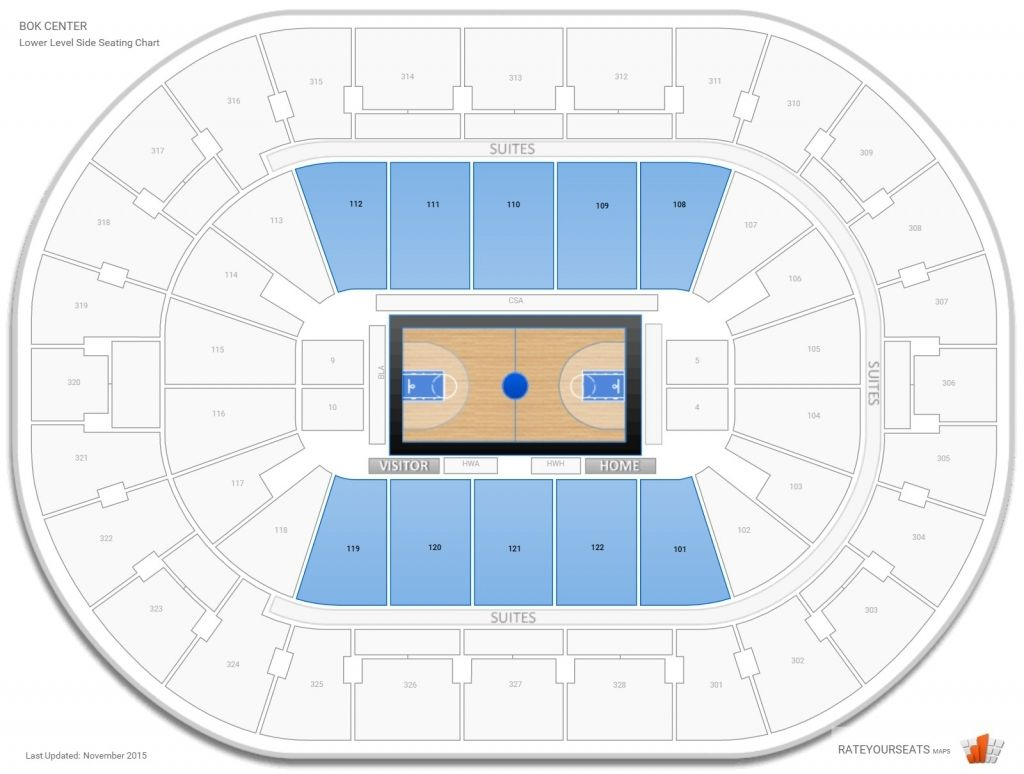The image depicts a detailed seating chart for the lower level of the BOK Center, highlighting side seating arrangements. The centerpiece of the map is an oval-shaped stadium with a gray outer boundary. Surrounding the oval are a series of numbered squares and rectangular shapes, indicating various seating sections.

Encircling the oval at a level just below the top and near the bottom are additional sections labeled "suites," which extend around the right side as well. At the very heart of the stadium lies a rectangular basketball court, which is brown with a prominent blue circle at its center. The court features two goals on either side, both marked by a blue center circle and circular interior area, representing the inside court.

Above and below the basketball court are blue-colored sections which appear to be designated seating areas. Notably, the seating near the bottom of the court is labeled "visitor" on the bottom left and "home" on the bottom right, indicating the respective team areas.